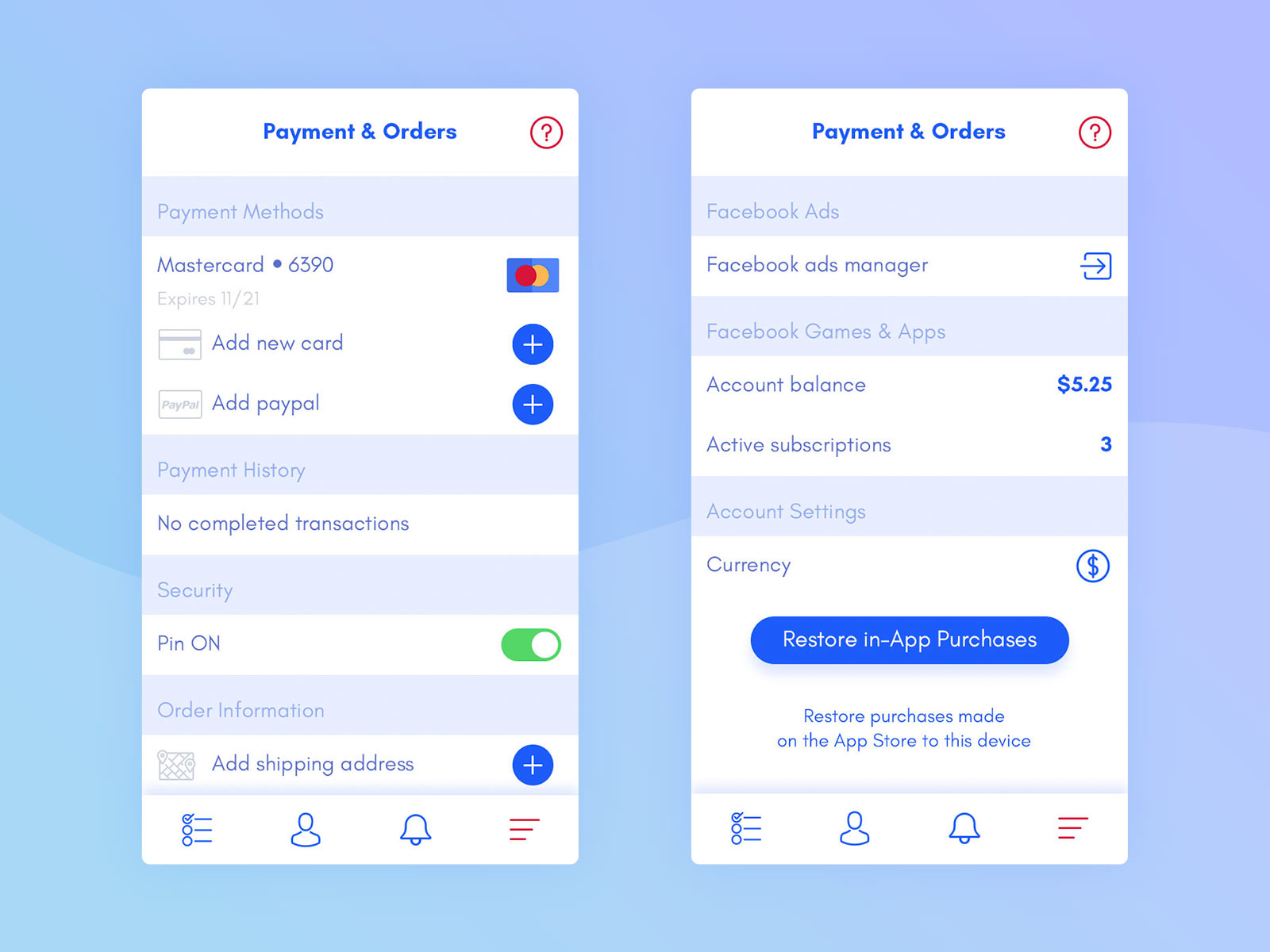The image features a user interface screen for managing payments and orders. The background transitions from lavender in the top right corner to a light blue color. Two primary sections are visible, separated by rectangles.

On the left side, the blue rectangle is labeled "Payments and Orders." Below it, there's a circle with a light gray interior and a red question mark, encircled by a red border. The text inside this section reads "Payment Methods" in gray, followed by "MasterCard 6390" in a purplish color, and "Expire 11-21" in gray. Other options include "Add New Card," "Add PayPal," and "Payment History" in gray, transitioning back to light gray background. The section concludes with "No completed transactions" in purple, and "Security" in purple as well.

To the right, there is another section beginning with "Order Information" and an option to "Add Shipping Address," indicated by a blue circle with a plus sign. This side mimics the "Payments and Orders" layout but includes additional elements like "Facebook Ads," "Facebook Ad Manager," "Facebook Games and Apps," and "Account Balance" displayed as $5.25 in blue. It provides an option to "Add to Subscription" and lists "Account Seven" as "Currency" with a blue dollar sign. Finally, a blue oval with white text reads "Restore in-app purchases," instructing users to restore purchases made from the App Store to their device.

The overall design is aesthetically light with soft pastel colors and clear, organized sections for an intuitive user experience.